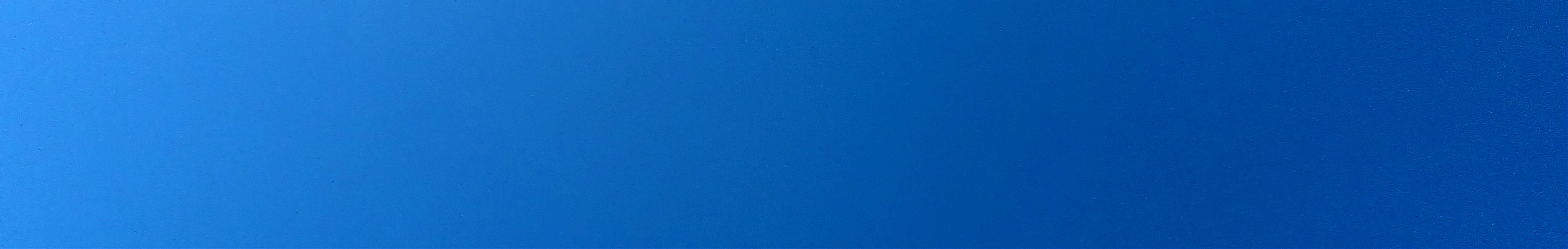The image depicts a simple, rectangular, horizontal bar with an approximate width of two inches and a height of half an inch. The bar has a subtle yet visually appealing gradient, transitioning from a light blue on the left side to a richer, darker blue on the right. This gradual shift in shades of blue evokes a sense of the sky just after dusk. The simplistic yet elegant design resembles a typical website banner ad but without any text or additional graphics, highlighting the beauty of the gradient itself.